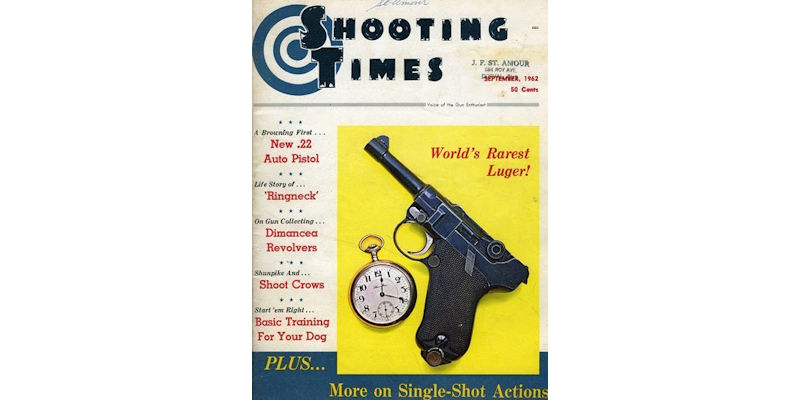This image depicts the cover of a classic or antique magazine titled "Shooting Times." The cover features a variety of vibrant colors, including white, black, blue, red, gray, yellow, and gold, which are well-positioned and spaced out. In the top left corner, there is a blue bullseye target. The title "Shooting Times" is prominently displayed at the top center, overlapping the bullseye slightly.

On the right side of the cover, a gun is positioned diagonally with its barrel pointing toward the top left corner. Below the gun's trigger, a pocket watch-style stopwatch is visible on a yellow background. The cover text includes headlines such as "World's Rarest Luger," "New .22 Auto Pistol," "Ring Neck," "Demacia Revolvers," "Shoot Crows," "Basic Training for Your Dog," and "Plus More on Single Shot Actions." Additional text is arranged along the top, left side, and bottom of the cover.

Overall, the image exudes a sense of meticulous organization, making it clear that it’s the front cover of an old magazine, likely focused on firearms and shooting activities.